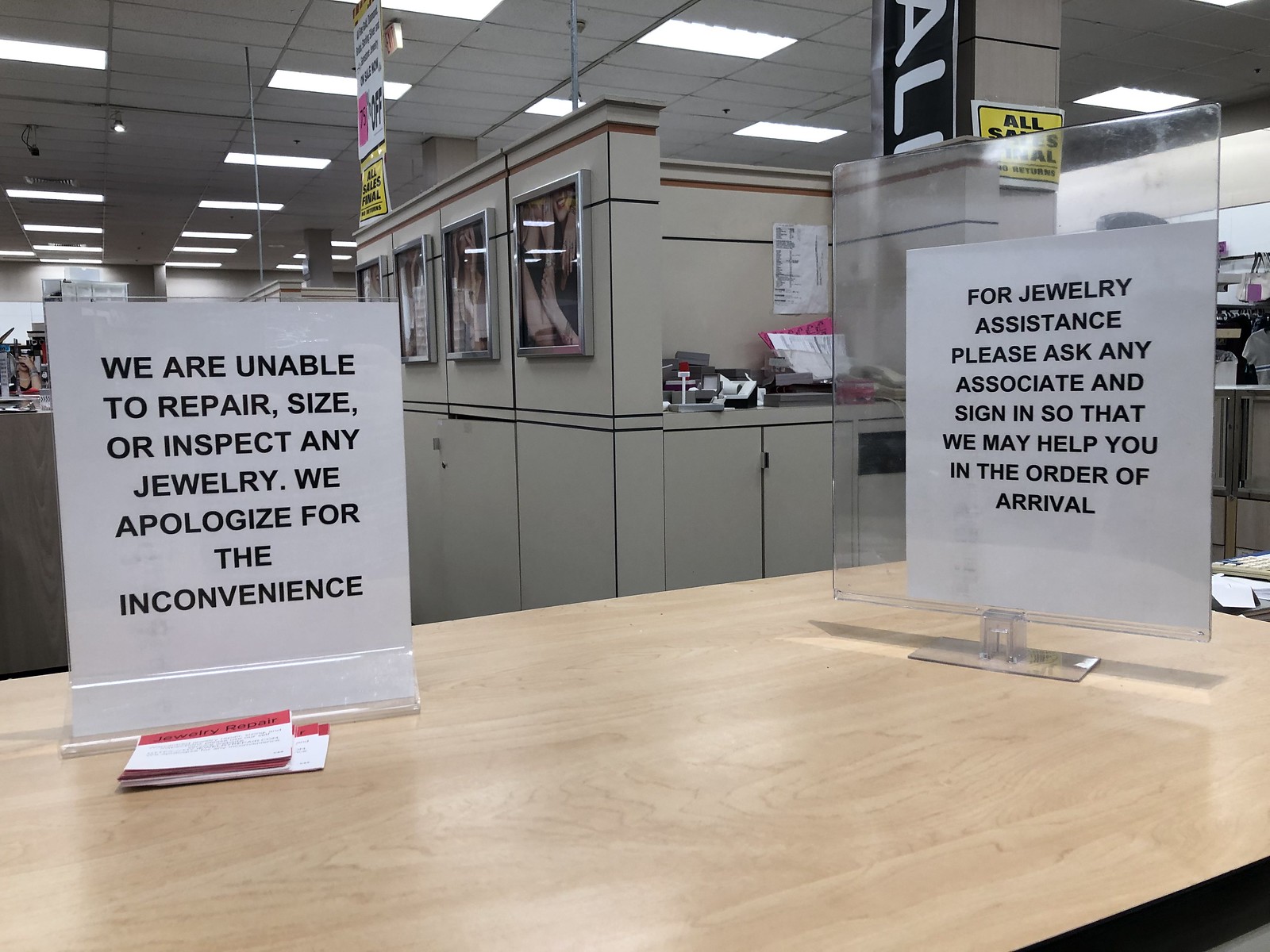This photograph depicts a corner of a department store, specifically showcasing a jewelry counter. The scene is bathed in the light from overhead recessed fluorescent fixtures embedded within a drop ceiling composed of tiles in a metal grid. Dominating the right side of the image is a gray column adorned with a prominent black, white-lettered sale sign running vertically. Attached to the front of this counter, which features a pale wood-colored laminate finish, are two clear plastic-framed signs: the first sign communicates, "We are unable to repair, size, or inspect any jewelry. We apologize for the inconvenience," while the second sign instructs, "For jewelry assistance, please ask any associate and sign in so that we may help you in the order of arrival." At the base of these signs sits a stack of white business cards edged with a red border.

In the background looms a gray cubicle-like structure, adorned with four thick-boxed, silver-framed images whose details are indiscernible, hanging in a row. Below these frames, the cubicle wall only reaches three-quarters of the height up to the ceiling, creating an incomplete partition. Additional details include a separate counter laden with various items, possibly including jewelry stands and a calculator with a roll of paper. A white paper with black text, along with other documents, decorates the wall above this counter. Although no people are visible in this tranquil scene, the array of details suggests a bustling environment typically aimed at customer service within a retail setting.